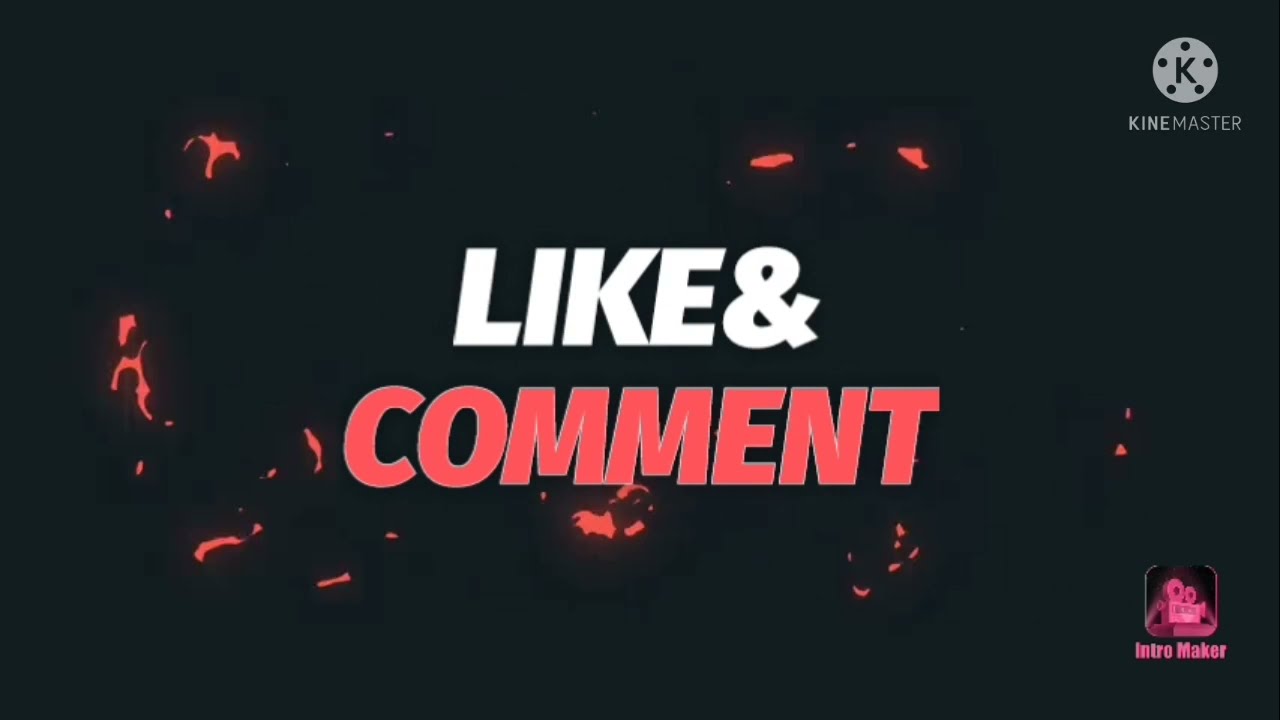The image features a striking design with a predominantly black, somewhat gray background, accented by dynamic, glowing red splotches that give it a fiery appearance. Central to the composition is large, all-caps text: "LIKE & COMMENT," where "LIKE &" is in white and "COMMENT" in bold red. In the upper right corner, there is a circular KineMaster logo— a 'K' encircled by five dots— with "KINEMASTER" written beneath it in white, with 'KINE' emphasized in bold. Additionally, the bottom right corner contains the text "INTRO MAKER," likely crediting the recording software used. The overall look suggests the image is a screenshot from a video, highlighting interactive prompts and the tools used in its creation.